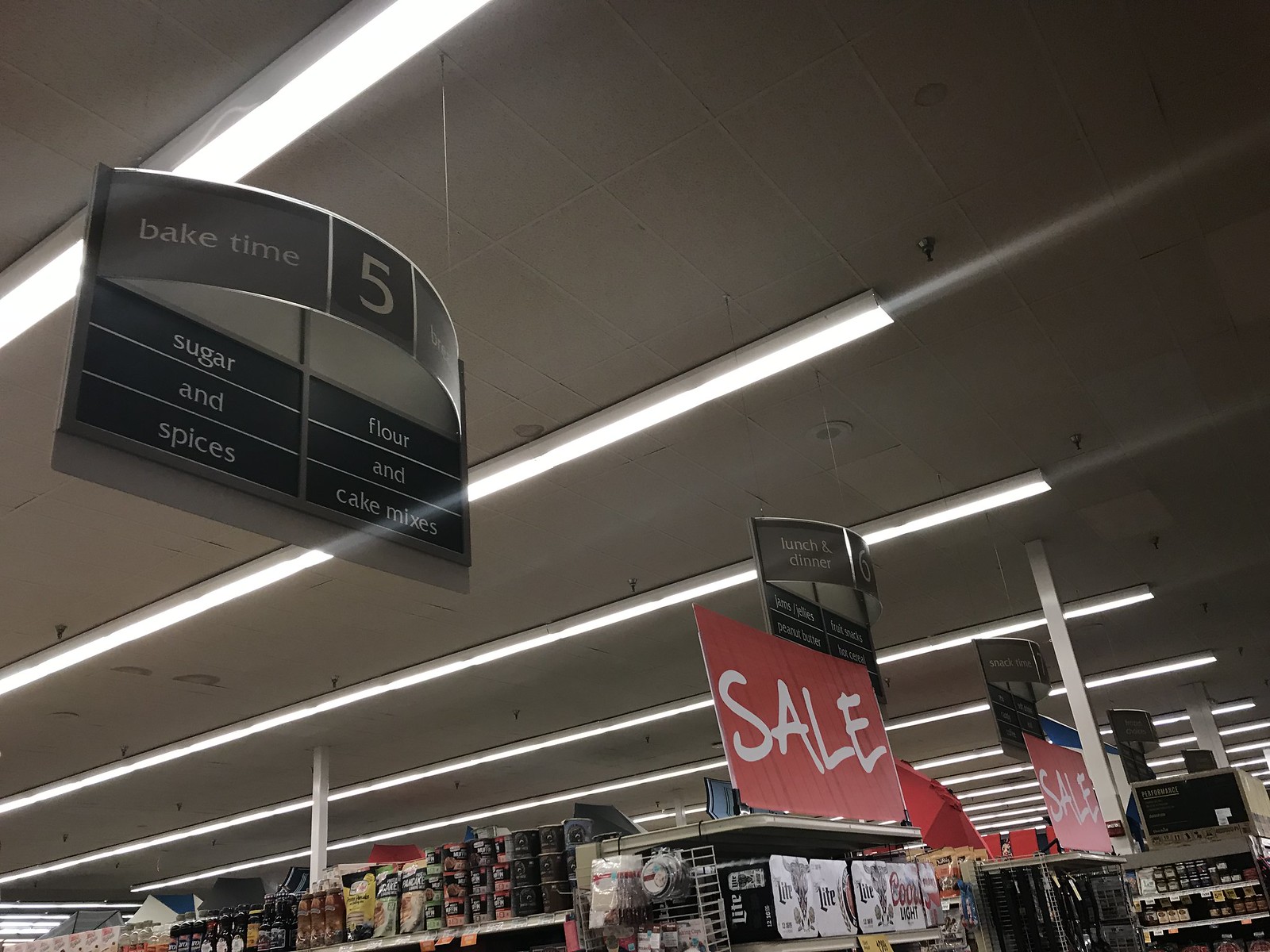This image captures the interior of a retail store, focusing on the ceiling and the signage indicating various aisles. The ceiling is comprised of typical gray office tiles adorned with long, illuminated strips of fluorescent lights. Below, several black signs with metal trim are suspended over each aisle, displaying the aisle numbers and their respective categories. Prominently in the foreground is aisle 5, which features signs labeled "Bake Time" on one side and "Bread" on the other. Within this aisle, the shelves are stocked with baking essentials including sugar, spices, flour, and cake mixes. The top shelf is visible, showcasing canisters of honey, jams, and what appears to be syrup.